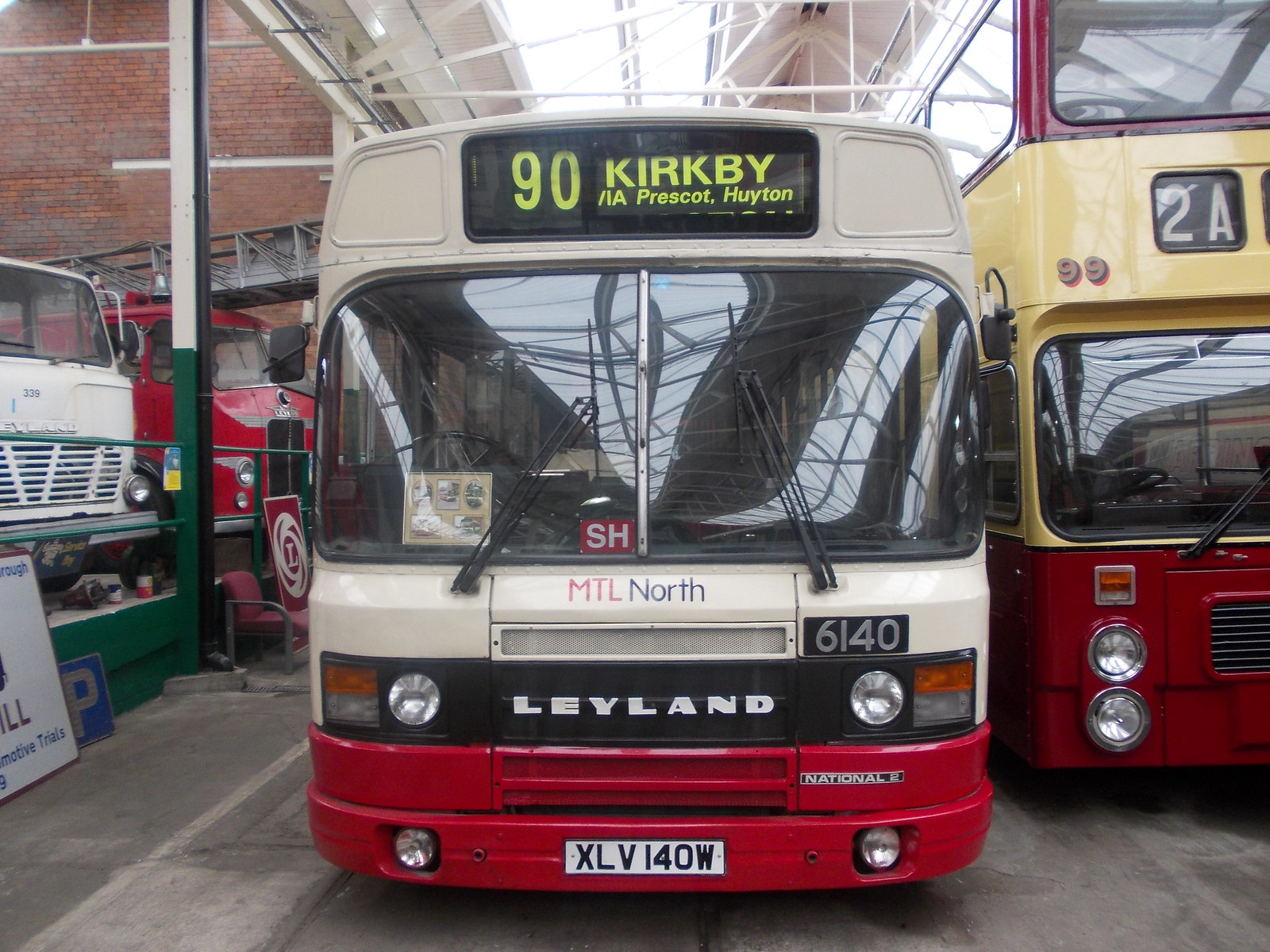A photograph of a bus station featuring predominantly buses. Central to the image is a single-decker bus marked with several distinct details: its red bumper with a white license plate displaying the number XLV14W, and a black grill with "LEYLAND" written in white letters. On the red bumper's right side, a black triangle contains a rectangle that reads "NATIONAL 2" in white letters. Above the right headlight is the number 6140 in gray letters. Centrally displayed above this are the letters "MTL" followed by the word "NORTH." On the windshield, there's a sticker with "SH" on a red background. The windshield, split into left and right sections, shows significant reflections and has windshield wipers pointing in opposite directions. The top section of the bus, cream-colored, features a black sign displaying "90 Kirkby VIA Prescott, Huyton" in white text. Surrounding this bus, several vehicles are parked: another bus to the right and some others in storage on the left. The setting appears to be a bus station or garage, with evidence of metal scaffolding overhead and sunlight filtering through. The location is framed by a brick wall to the left and includes a mix of single-decker and double-decker buses, one identifiable with a "2A" marking.